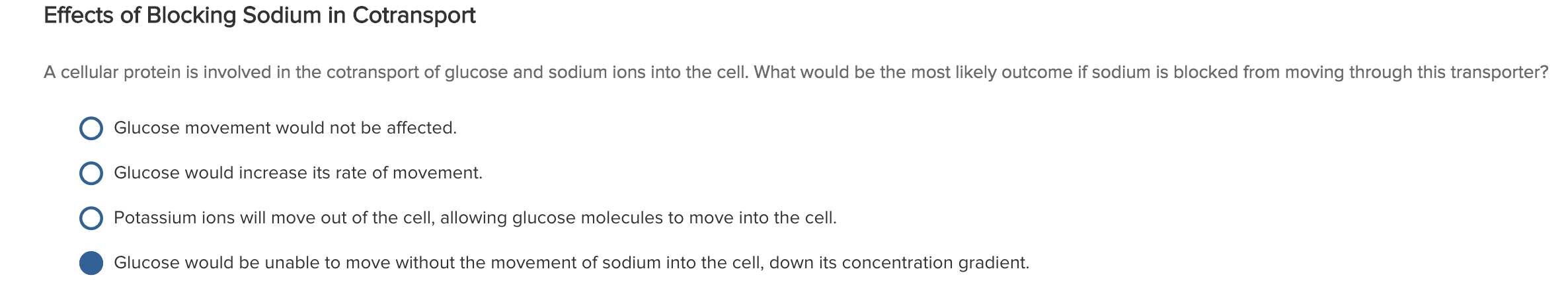**Image Description:**

The image features a multiple-choice question interface set against a completely white background. The text in the upper left corner serves as the title of the question, stating: "Effects of Blocking Sodium in Cotransport." Below the title, there is a clear space followed by the question. The question reads: "A cellular protein is involved in the cotransport of glucose and sodium ions into the cell. What would be the most likely outcome if sodium is blocked from moving through this transporter?"

Following another space, five answer choices are listed:

1. Glucose movement would not be affected.
2. Glucose would increase its rate of movement.
3. Potassium ions will move out of the cells.
4. Glucose would be unable to move without the movement of sodium into the cell down its concentration gradient. (This option is selected)
5. There are no additional answer options listed.

The selected answer is clearly indicated, suggesting that the blocking of sodium would prevent glucose from moving due to its reliance on the sodium concentration gradient for transport into the cell.